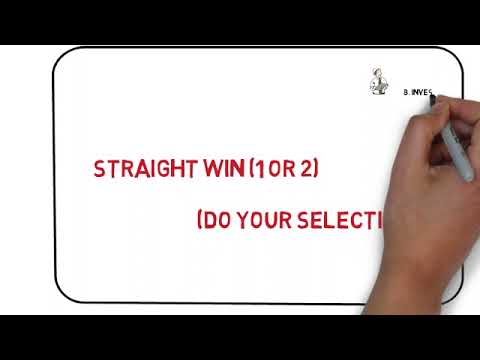The image is a horizontally rectangular screenshot, bordered by thick black bars on the top and bottom. Within this frame, a smaller black-bordered whiteboard occupies most of the image. The focal text, written in bold red lettering across the center of the whiteboard, reads "STRAIGHT WIN - 1 OR 2 - (DO YOUR SELECTION)." On the far right side, a human hand, possibly of tan complexion, is holding a black Sharpie and writing the letters "B-I-N-V-E-S." Nearby, to the left of this writing, there is an indistinct drawing of a person. The image appears to be from a tutorial or instructional video, guiding viewers through a specific process, although the exact details are unclear.